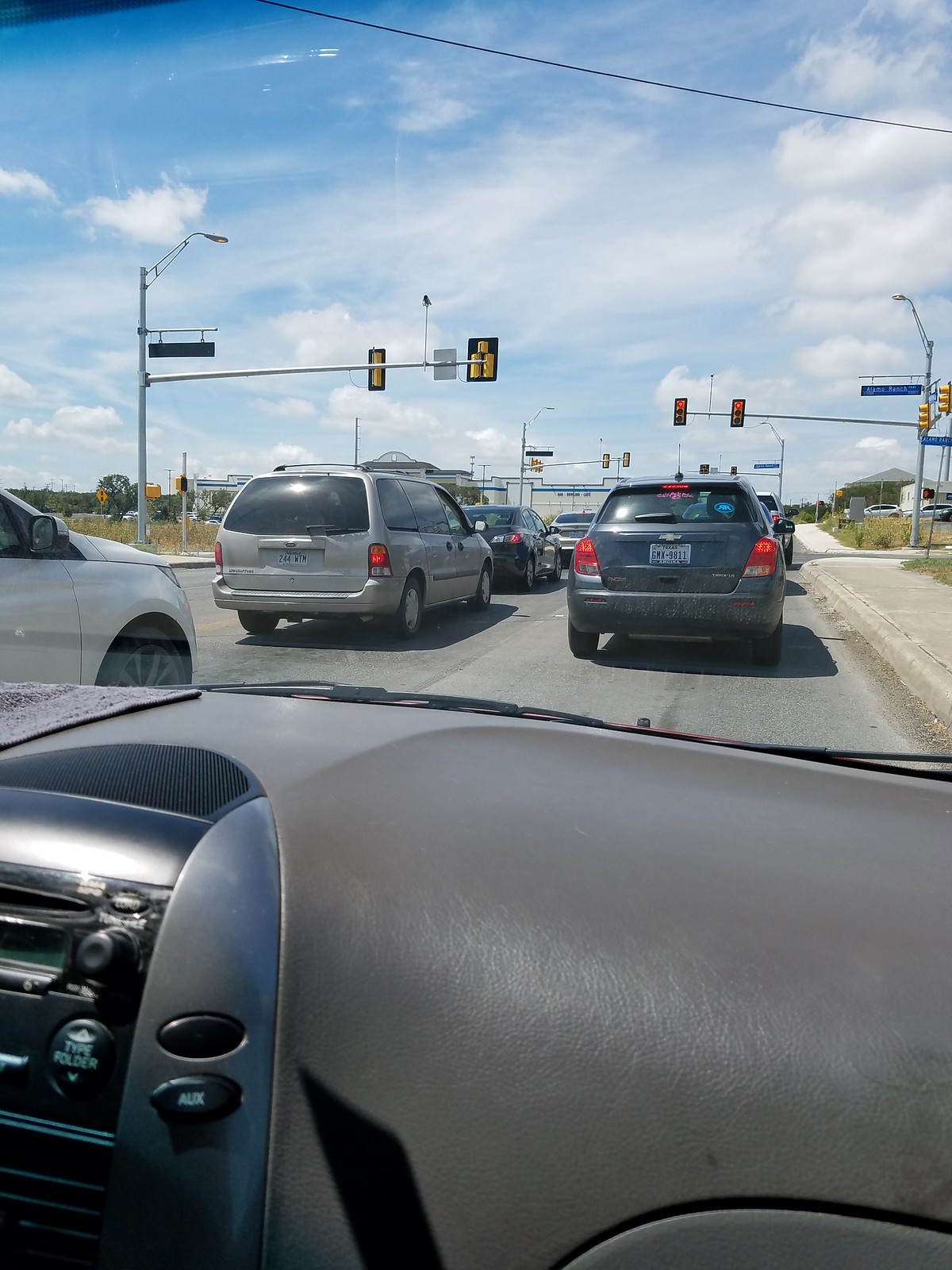The photograph, taken from the passenger seat of an older vehicle, captures a bustling scene on a city street during daytime. The dashboard, a dark gray with silver radio details, suggests a car from the early 2000s. Through the windshield, we see a red stoplight holding up traffic on a broad two-lane road. Directly ahead is a gray car, with a white car, a gray sedan, and a dark minivan all lined up in the left lane. The right side of the image features a deserted sidewalk that runs alongside the road. In the distance, tall brown grass and indistinct business buildings punctuate the open landscape. Above, the sky stretches out in a bright blue expanse, dotted with both fluffy and wispy clouds, adding a sense of openness to the scene.